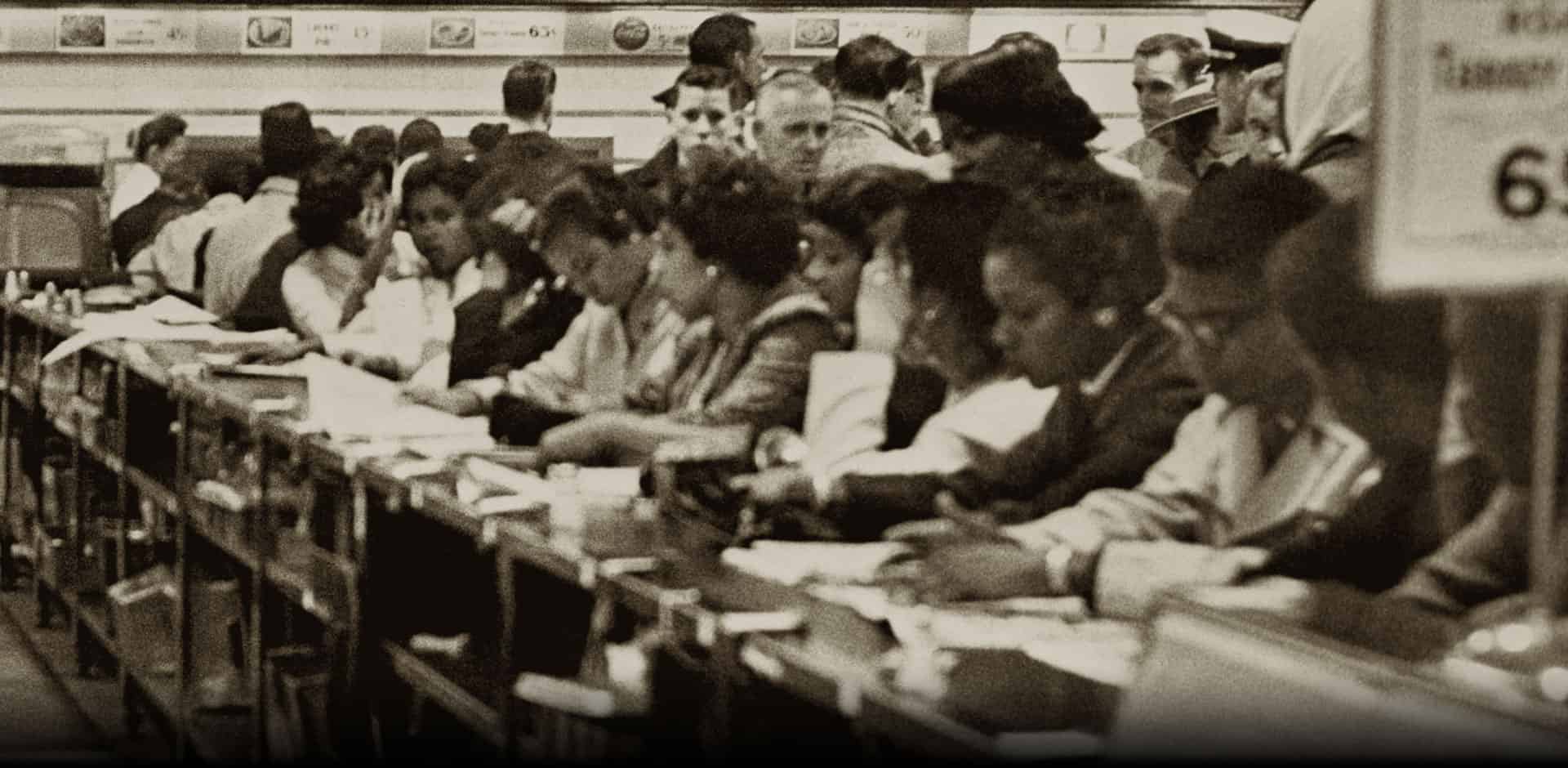This is a black-and-white photograph from the late 1950s or early 1960s that captures a significant moment during the Civil Rights Movement. The image is wider than it is tall and shows a long row of African-American students, both male and female, sitting at a lunch counter. They appear to be engaging in a peaceful protest, studying and reading from their books, with papers laid out in front of them. There are perhaps 15 to 20 individuals lined up, some wearing glasses and earrings, all seated elbow to elbow. Behind them, several white men, including some wearing hats, are visible looking at the students with expressions of anger and hostility. The setting seems to be a dining hall, as evidenced by a menu sign on the wall that includes items priced at 65 cents. Additionally, there are police officers in the background, suggesting that an arrest might be imminent. This poignant image vividly illustrates the tension and courage during the era of racial segregation and the fight for equality.